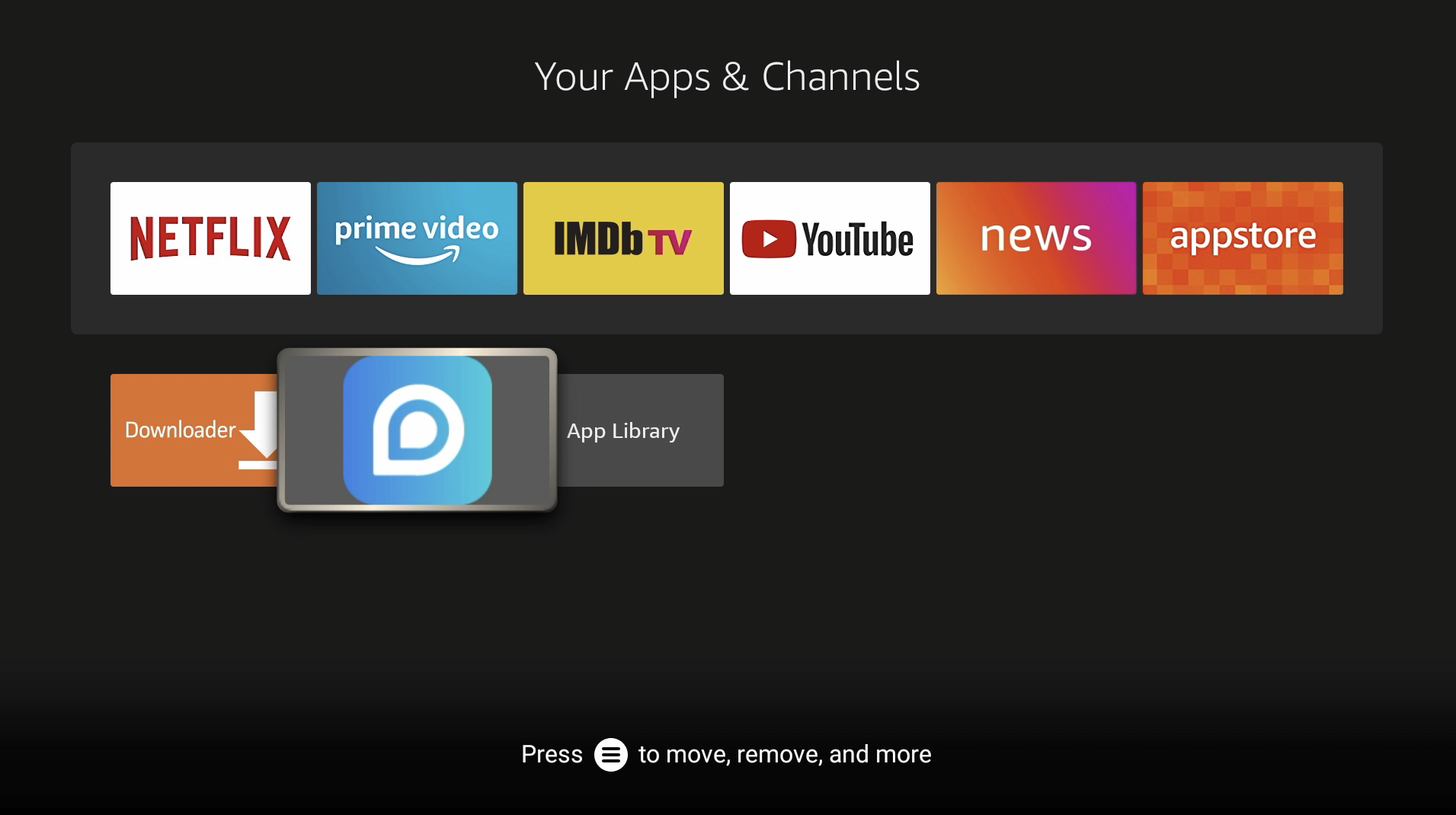The image is a screenshot of an application page featuring a black colored background. At the top center of the screen, white text reads, "Your Apps and Channels." Below this heading, there are several icons representing various news channels and online video services. From left to right, the icons are as follows: 
1. Netflix, depicted with red text on a white background.
2. Prime Video, featuring white text and a white curved arrow against a blue background.
3. IMDB TV, displayed with black and red text on a yellow background.
4. YouTube, illustrated with a red and white play button icon on a white background.
5. Neal's, shown in white text on a gradient background of pink, orange, and light purple.